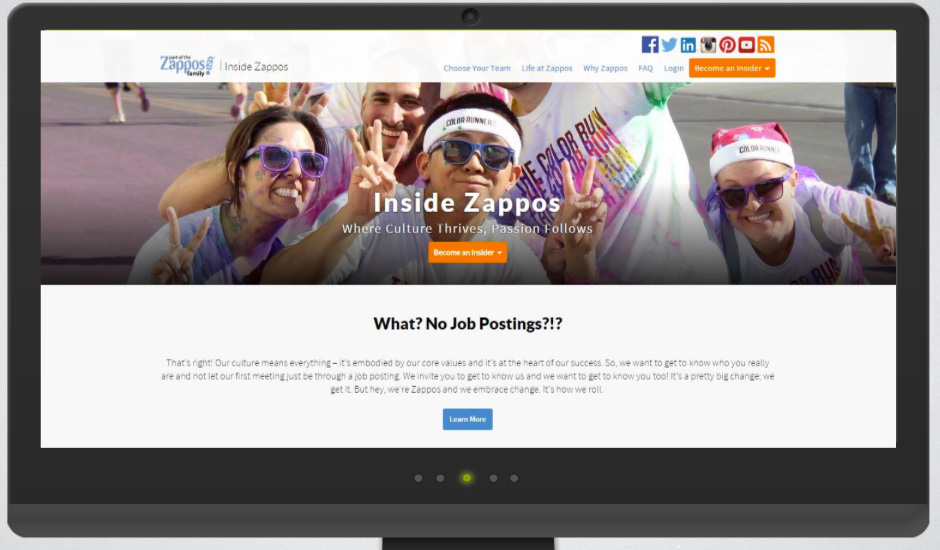The image showcases a computer monitor with a sleek black trim. At the bottom of the monitor, there are five small dots, with the center dot illuminated in a fluorescent lime green, which likely represents a power or status light. The web page displayed on the monitor has a white background and a white top banner. The banner prominently features the text "Zappos Family," followed by navigation options towards the right: "Choose Your Team," "Life at Zappos," "Why Zappos?," "FAQ," "Login." Additionally, there's an orange banner that says "Become an Insider" in white text, accompanied by a drop-down menu.

Above the banner, there are icons for various social media sites, including Facebook, Twitter, Instagram, LinkedIn, Pinterest, and YouTube. The background image on the page depicts an outdoor scene where a group of people, wearing t-shirts, sunglasses, and headbands, are huddled together and smiling. Some individuals are showing peace signs. A street is visible behind them, with people running.

The main text on the webpage reads, "Inside Zappos: Where Culture Thrives & Passion Follows." Below this, there is another orange banner with a drop-down menu, again stating "Become an Insider." Further down, it mentions there are no job postings with the text, "That's right, our culture means everything." There is additional text that is difficult to read, followed by a call-to-action button that says "Learn More" in a blue square with white print.